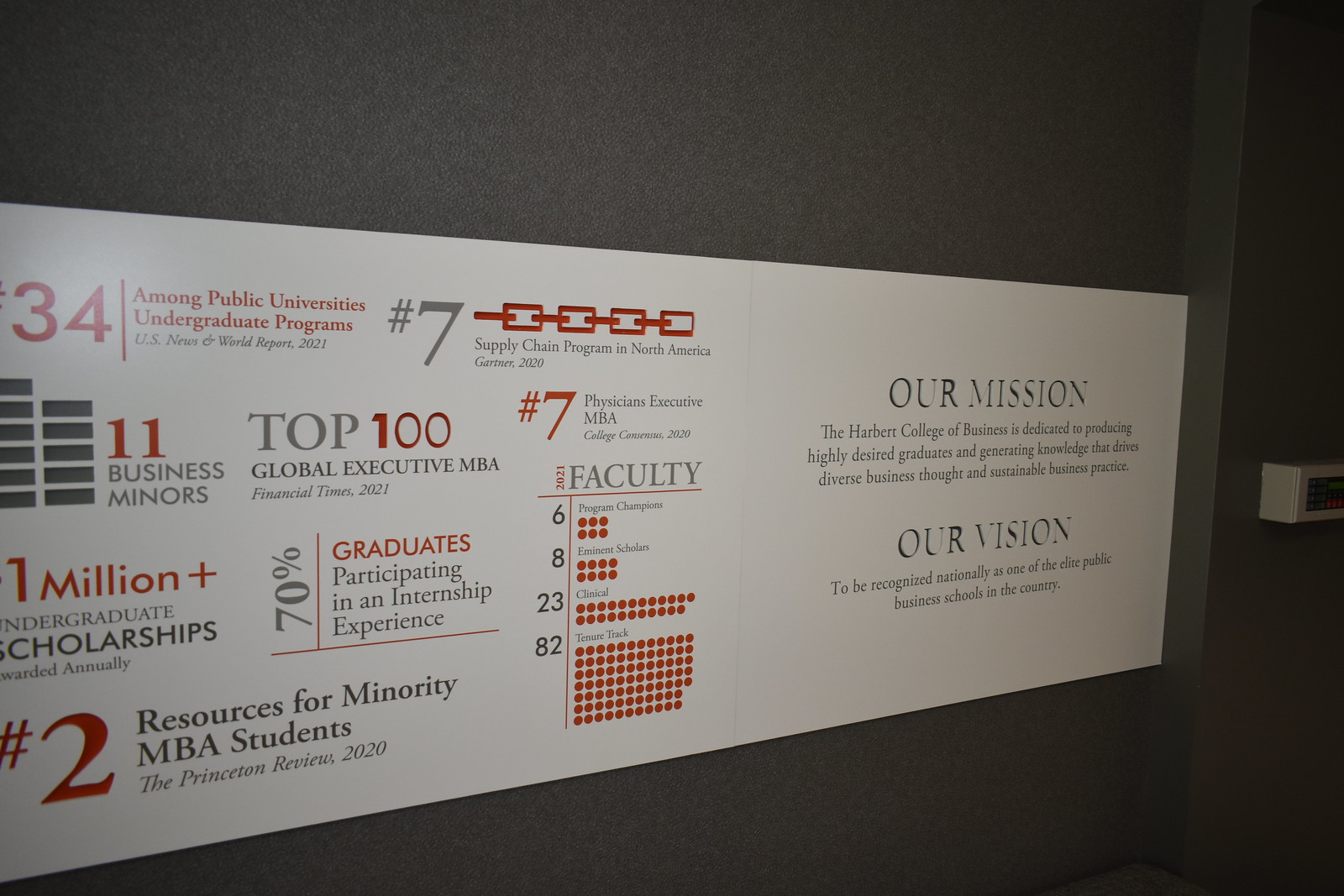This color photograph, taken indoors in a landscape orientation, captures a university display centered on a dark gray wall. Dominating the scene is a broad, white horizontal banner running almost the width of the image, adorned with red and black text. To the far right of the banner are the university's mission and vision statements. The mission reads: "The Harvard College of Business is dedicated to producing highly desired graduates and generating knowledge that drives diverse business thought and sustainable business practices." The vision states: "To be recognized nationally as one of the elite public business schools in our country."

Scattered across the banner are various accolades and statistics: "34 among public universities undergraduate programs," "Number seven supply chain program in North America," "Top 100 global executive MBA," "Number seven physicians executive MBA," "1 million plus undergraduate scholarships awarded annually," "Number two resources for minority MBA students," "70% graduates participating in an internship experience," and faculty numbers including "six program champions, eight eminent scholars, 23 clinical, and 82 tenure-track."

The banner features graphs, such as a black-bar graph indicating "11 business minors" and another detailing faculty statistics. Positioned to the far right of the image is a white thermostat, contrasting against the dark background. The photograph's realistic style underscores the university's achievements and aspirations.